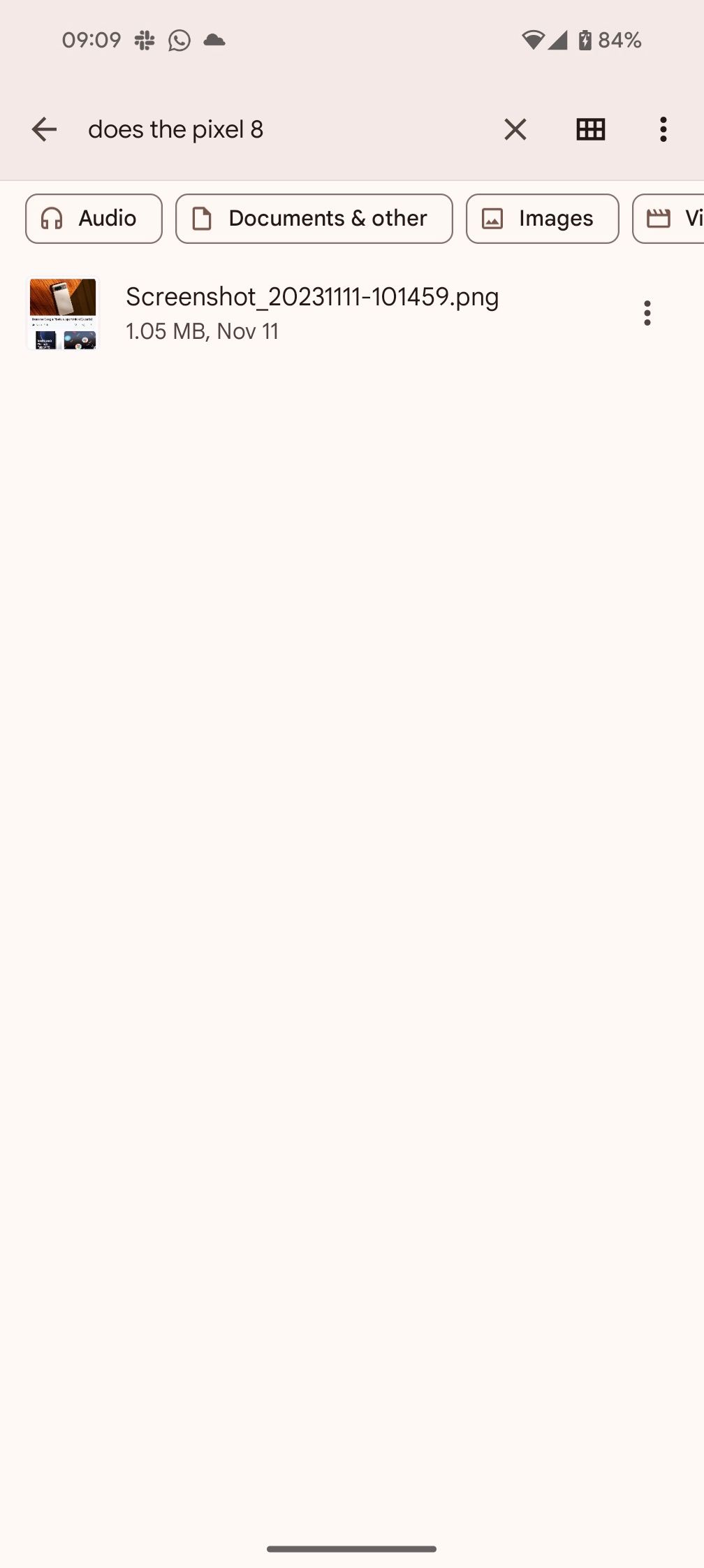This image depicts a cell phone screen displaying a webpage with minimal content. The screen, oriented vertically, features common cell phone indicators in a faded red color at the top. The time is shown as 09:09 on the left, with three icons to the right indicating open apps or options: a cloud app, a speech bubble with a telephone inside, and a cross symbol. 

To the left, various cell phone indicators are presented from left to right, starting with the Wi-Fi strength, followed by a triangle indicating cell reception, and a battery icon showing 84% charge remaining.

Below the indicators, the screen shows an option labeled "Does the Pixel 8" with a left arrow, suggesting navigation to a previous screen. On the right, there is an 'X' icon for closing out, followed by a rectangle with six white dots, the function of which is unclear, and vertical three dots indicating more options.

The main portion of the screen is largely blank, but there are several categorized buttons below the title, each represented by icons: audio with a headset icon, documents with a page icon, images with an image icon, and a partially visible video option showing a clapperboard icon with the letters "VI".

A particular file is highlighted under these options, identified as a screenshot named "screenshot_20231111-101459.png", indicating it is a PNG image file. The image is presumably of a cell phone with other images on it, occupying 1.05 megabytes and recorded on November 11th. To the far right of this file are three dots signifying additional actions for managing the file.